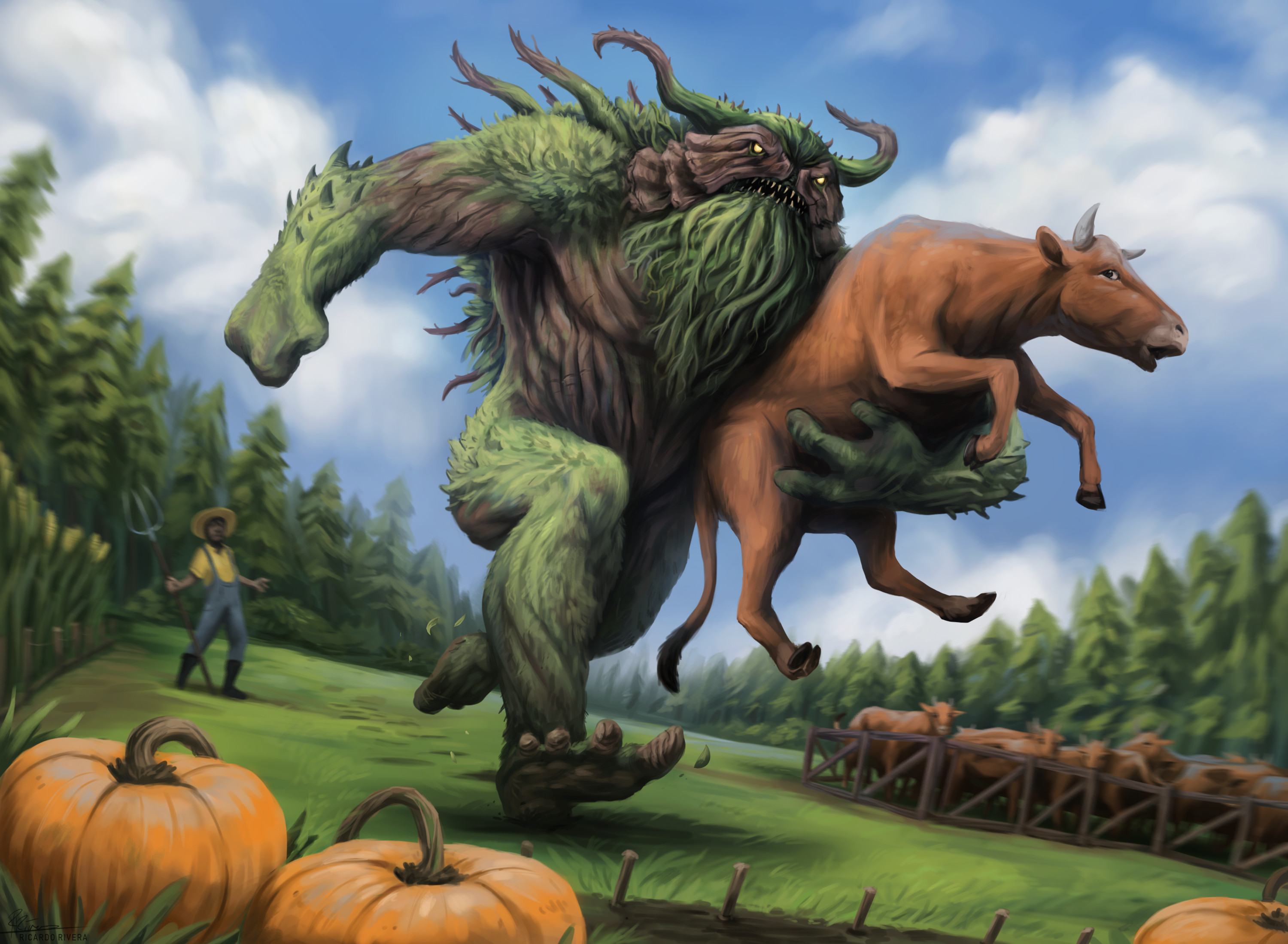In this whimsical and mythical scene, the foreground is adorned with pumpkins—two fully visible on the left and partial ones at the corners on the right. A lush grassy meadow stretches out in the center, flanked by dense, forested woods that converge at the back of the image. On the right side, before the trees, stands a pen containing cattle, their presence adding a rustic charm to the setting. 

On the left side, a small farmer dressed in a yellow shirt, blue trousers, and braces is depicted, his facial expression one of shock. The reason for his astonishment is the surreal sight occupying the center of the image: a colossal green giant. The giant, an impressive figure, has four-toed feet and vibrant green limbs, but a more earthy brown central body. His face features two brown patches framing expressive eyes, a green beard cascading from his chin, and tendrils sprouting from his head and back, enhancing his otherworldly appearance.

In the giant's left arm is a distressed cow, its size relatively small compared to the giant’s enormous stature, almost covering his body up to his head. The scene captures the dynamic moment of the giant making his escape, while the farmer, arms outstretched, leans back in shock at the bizarre spectacle unfolding before him.